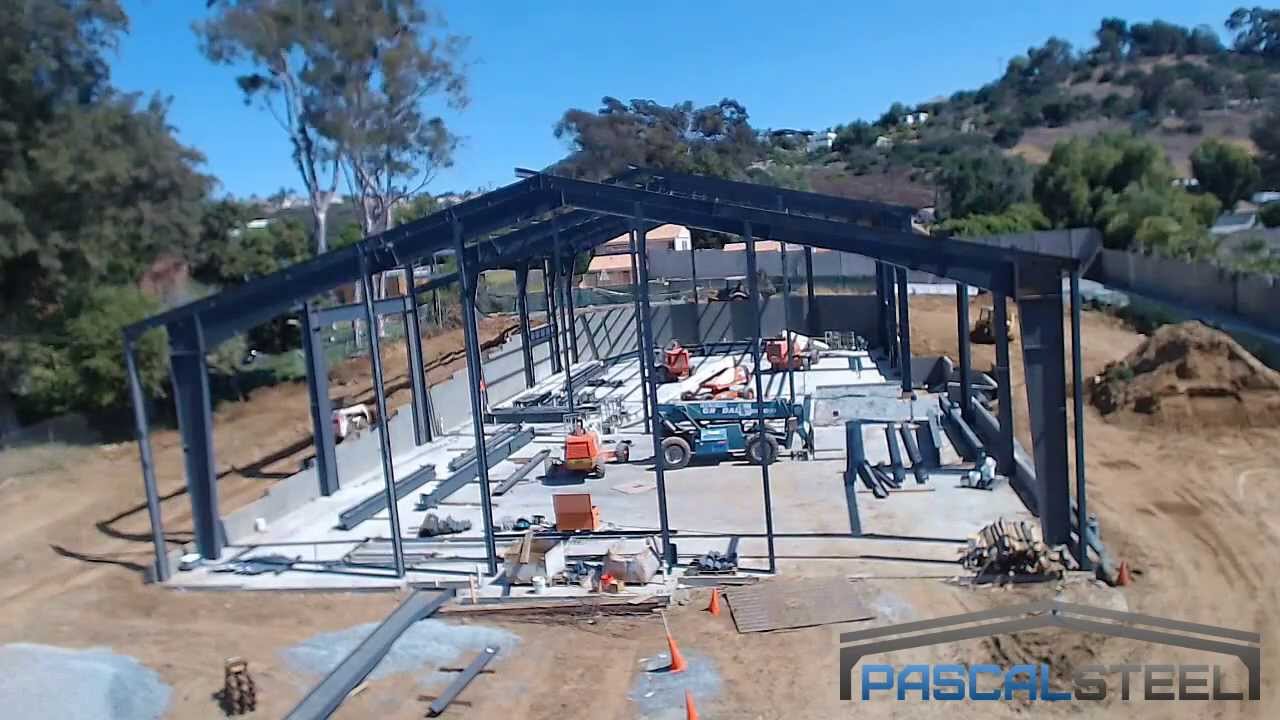The photograph captures an active construction site for what appears to be a commercial building by Pascal Steel, as indicated by the logo in the bottom right corner. The image prominently features the steel framework of the building, constructed with dark blue-gray metal beams and I-beams. The concrete foundation is already laid, and partial walls made of gray stone or concrete have started to go up along the left and back sides of the structure. The ground around the site has been cleared down to dirt, with a significant mound of dirt to the right. Scattered throughout the site are various construction vehicles, including a blue genie lift and several orange tractors, as well as steel beams and other building materials. Orange safety cones are positioned near the front of the building. The scene is set under a bright blue sky, with hills and green trees providing a picturesque backdrop. The absence of workers suggests they might be on a break, although equipment and materials indicate active construction.